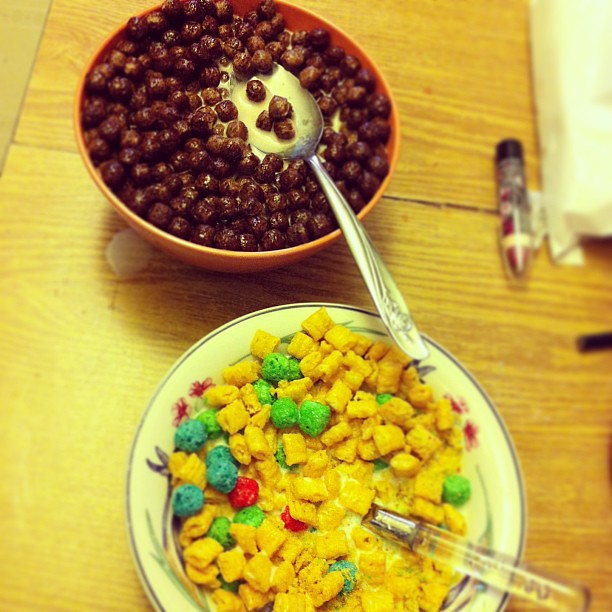This detailed color photograph captures an overhead view of two bowls of cereal positioned on a wide-planked, tan-colored wooden dining table. Near the bottom edge of the image is a white china bowl adorned with a gray rim design, containing a children's cereal mix of corn-colored squares and colorful blue, green, and red berry pieces. A clear lucite spoon with a partially visible metal base is placed at the 4 o'clock position within this bowl. Positioned towards the top center of the image is a clay-colored bowl filled with dark brown cocoa pebbles-like cereal, in which a silver spoon rests on the bottom right-hand side, its bowl containing milk and a few cereal pieces. In the top right corner of the image, partially out of frame, one can glimpse a book and a brown crayon adding an element of casual, lived-in detail to the scene. The tabletop's yellowish tint suggests a warm, possibly filtered lighting that casts a soft glow over the entire setting.